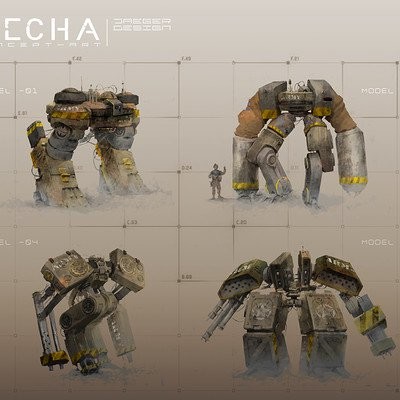The image depicts a design concept featuring four large, robotic figures arranged in a grid pattern against a gray background. Each figure is constructed from a combination of brown, silver, gray, black, and yellow mechanical components. The figures are identified with white text in the top left corner spelling "E-C-H-A" and labeled as Model 01-04-EL-EL, alongside other numeric indicators.

In the top left quadrant, there are notably large, robot-sized legs, forming what appears to be the lower torso of a larger structure, possibly with two people standing on or near it. The top right quadrant displays a complete figure with long arms, legs, and a short torso, standing next to a human figure for scale, emphasizing the robot's impressive size. The bottom left quadrant features a figure with two legs, square-like large shoulders, and mechanical arms designed to bend at the elbows. The final robot shown in the bottom right quadrant appears almost entirely complete, characterized by square shoulders, square legs, and arms equipped with three tubes on the left and a gear contraption on the right.

Despite varying degrees of completion and orientation, all the robots are constructed from the same materials, with some having visible weaponry. The human figure's presence provides a sense of scale, highlighting the robots' towering stature. The background appears monochromatic, and the mention of grass in the setting suggests it could be an outdoor scene.